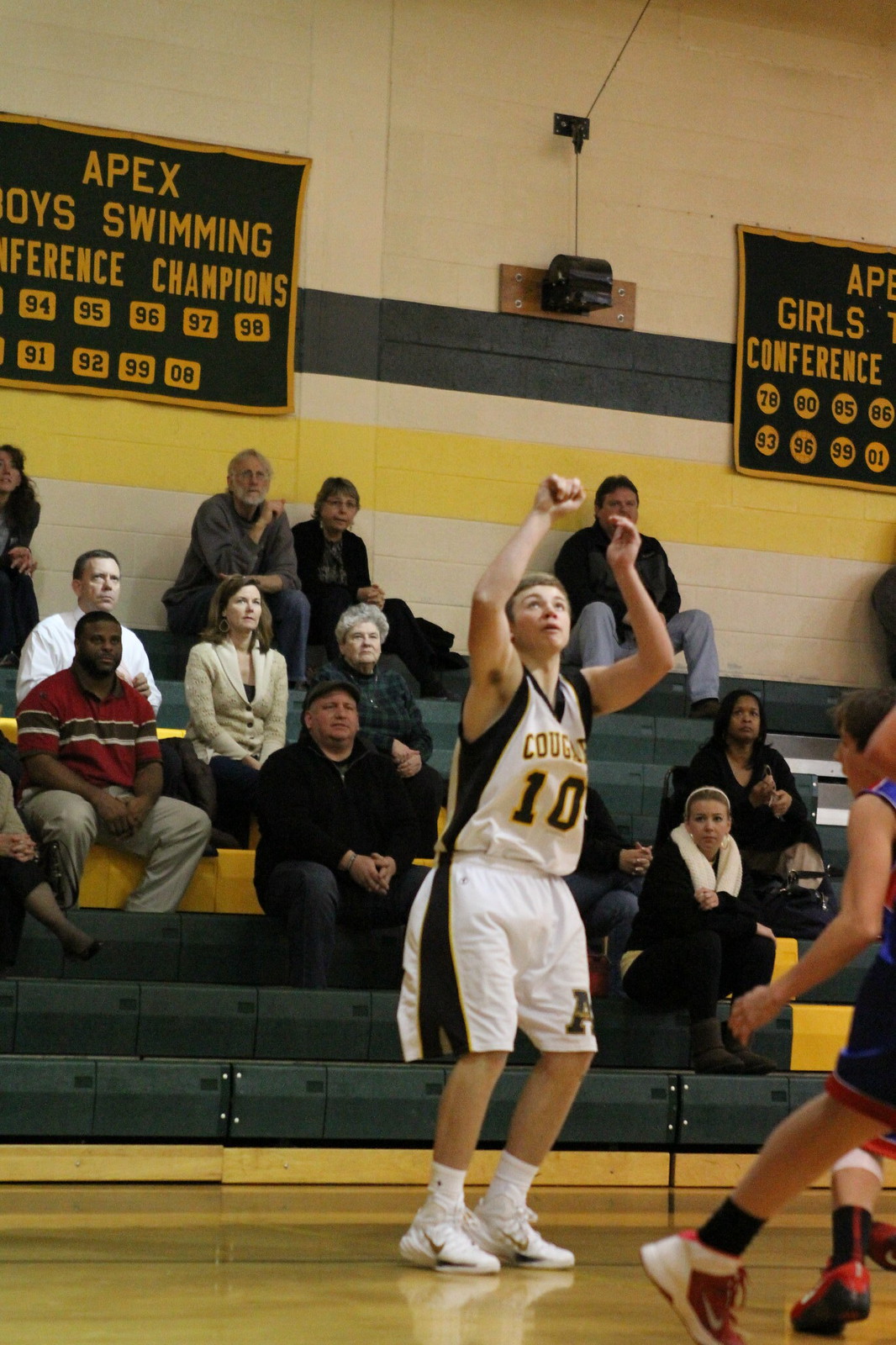This detailed image captures a high school boys' basketball game in progress, presumably in a gymnasium adorned with various banners. At the center of the action is a young player, number 10 of the Cougars, who appears to have just taken a shot, as indicated by his still-perfect shooting form. He is dressed in a white uniform with black side stripes on his shorts and jersey, which also features a gold accent and the letter 'A' on the left bottom of his shorts. His team wears white tennis shoes with a gold stripe, contrasting with their opponents' darker blue jerseys and shorts with black and red shoes. The background reveals a modest crowd of roughly a dozen spectators seated on wooden pull-out bleachers. Behind them, the gym's cinder block wall displays stripes in dark blue or black and yellow, along with banners celebrating achievements in boys' swimming and girls' conference championships, though parts of the banners are cut off in the image.